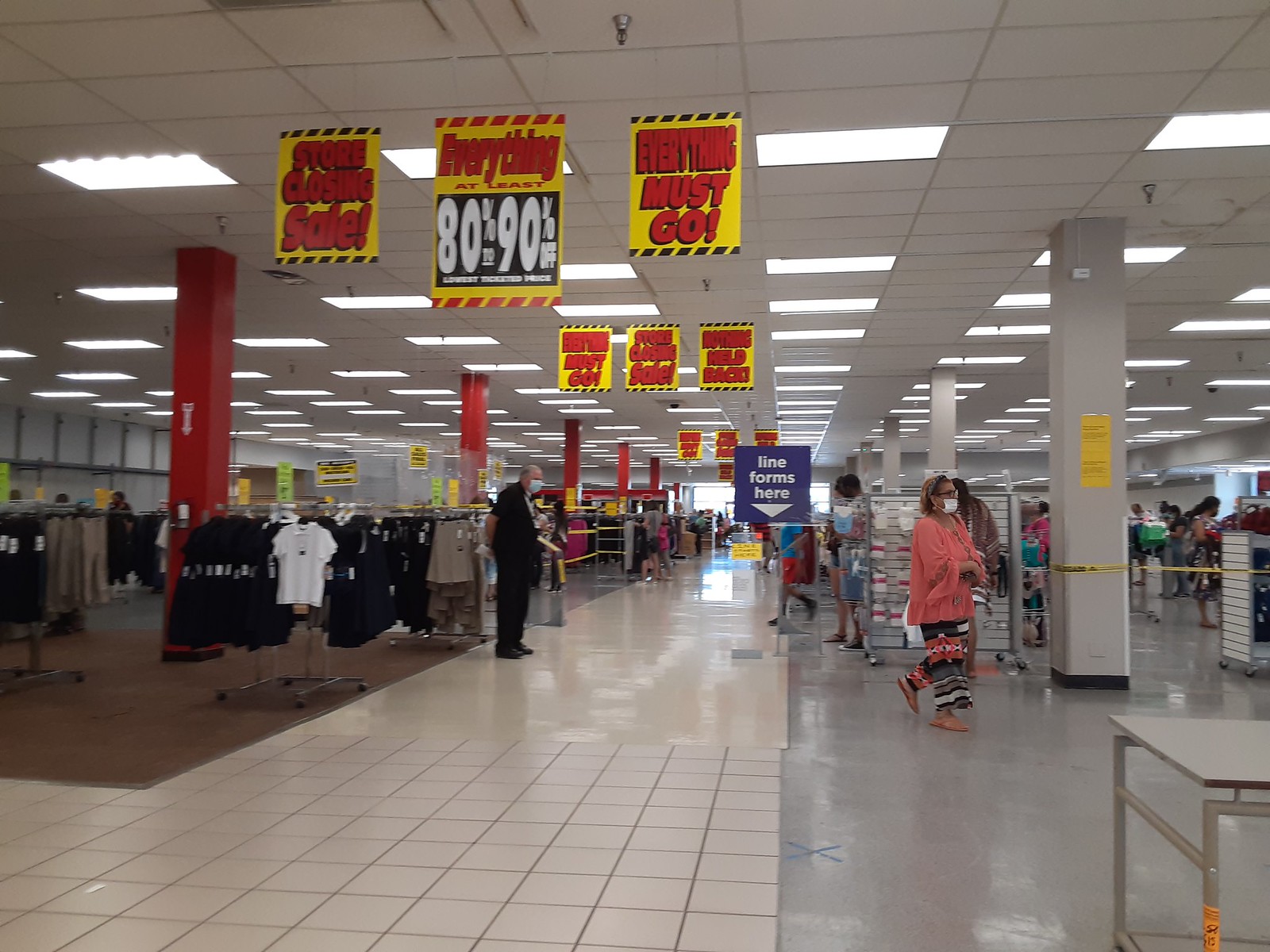This photograph captures the interior of a retail shopping center, specifically a department store, during its closing sale. The ceiling features a grid of white fluorescent lights that illuminate the spacious, open layout, punctuated by large, sturdy column posts. Suspended from the ceiling are numerous bright yellow signs proclaiming drastic discounts ranging from 80% to 90% off, accompanied by urgent messages declaring "Everything Must Go" and "Store Closing Sale," indicating the store's impending closure, likely due to going out of business. Several shoppers, all wearing masks—hinting that the photo was taken during the COVID-19 pandemic—traverse the store's aisles. On the left side of the image, various racks display t-shirts, skirts, and other garments available for sale in this final clearance event.